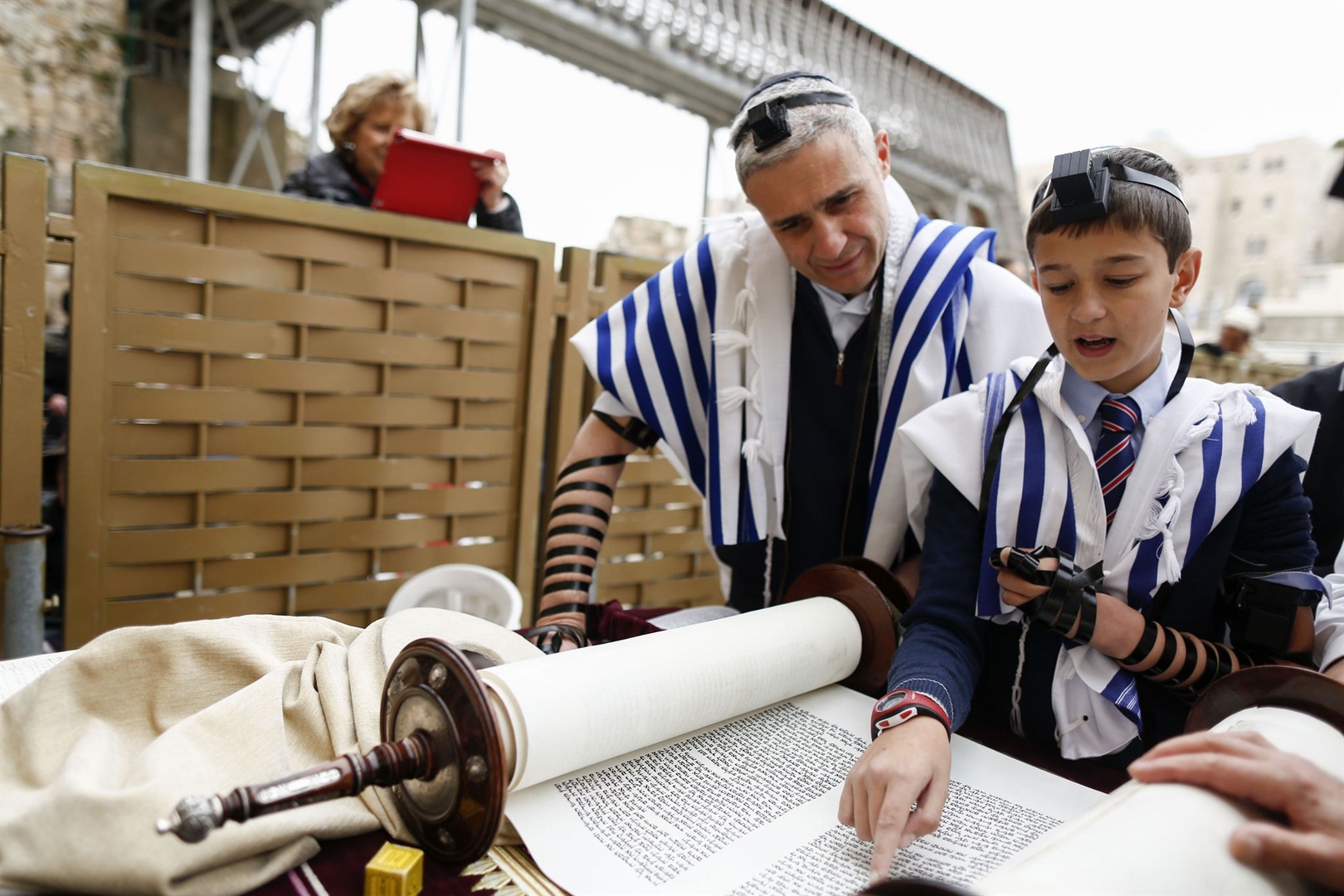In the image, a young Jewish boy and an older Jewish man are deeply engaged in reading from a large scroll. The boy, who appears to be in his early teens, is pointing to a specific passage and reading it aloud. He is dressed in traditional religious attire, which includes a blue and white striped shawl (tallit), a pin-striped tie, and a blue sweater over a white dress shirt. He has a red digital watch on his right wrist and a headband known as a frontlet (tefillin) on his head, with a leather strap wound around his arm.

The older man, standing closely behind the boy and looking over his shoulder, is similarly dressed in a white dress shirt, sweater, and a blue and white striped shawl. He also wears a frontlet and leather arm bindings, indicating his participation in ritual practices.

In the background, a wooden fence separates the main subjects from a slightly out-of-focus building. Over the fence, a woman can be seen holding a book, seemingly observing the two as they read from the scroll. Additionally, there's a hand resting on one of the scrolls in the foreground, suggesting the presence of another individual involved in the reading.